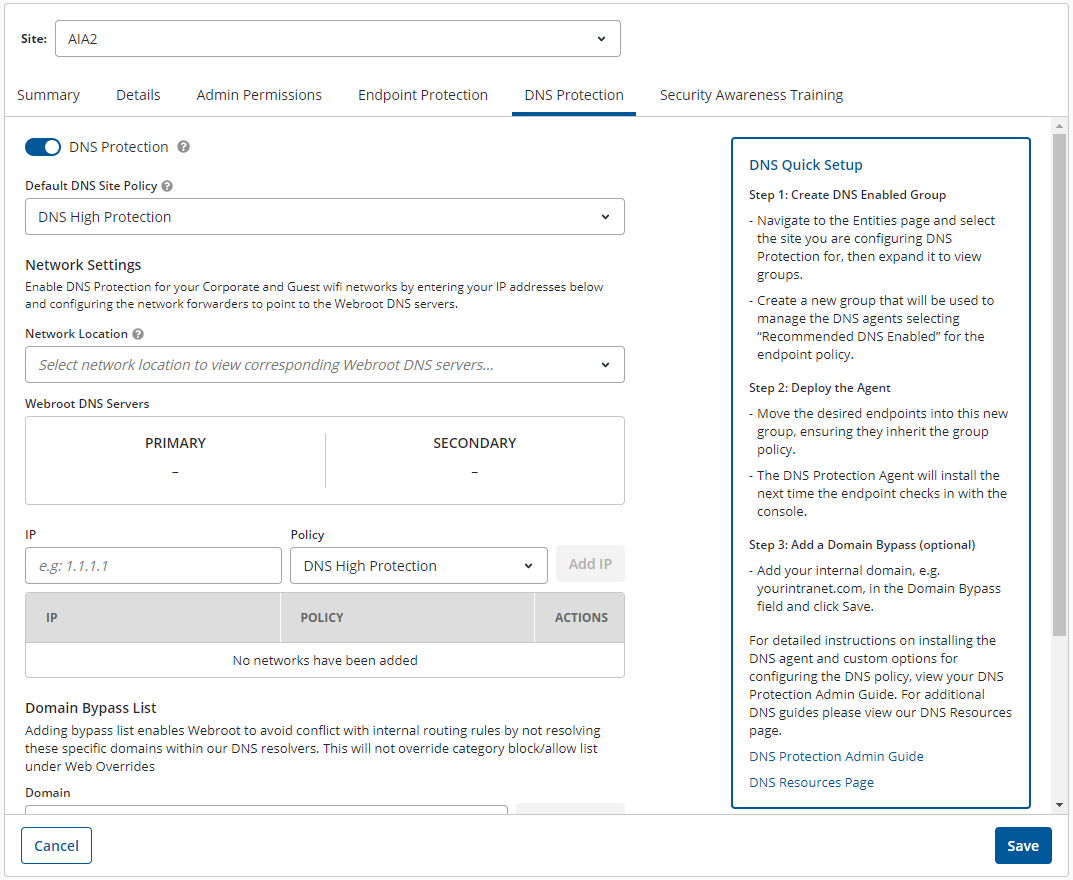The image depicts a complex interface with multiple sections and options. Here is a detailed description:

Starting at the top, there is a gray-outlined rectangle featuring a label on the upper left-hand corner. Below this label, within the rectangle, there is another gray-outlined rectangle with some words or numbers in it and an arrow pointing downward. This section appears to be labeled with the following categories: "Summary Details," "Admin Permissions," "Endpoint Protection," "DNS Protection," and "Security Awareness Training."

Under these categories, there is a gray dividing line, with a blue line running above it, specifically under "DNS Protection." To the right side, there is a button featuring a white circle and a label next to it, followed by a gray circle containing a question mark. Additional text follows, accompanied by another gray circle with a question mark.

Further down, there is yet another gray-outlined rectangle containing words and an arrow pointing downward, with more text below it. This section is followed by another labeled area, also framed by a gray-outlined rectangle with a question mark in it.

Continuing downward, there is a larger gray-outlined rectangle labeled "Primary" on the left-hand side, divided by a vertical line, with "Secondary" on the right-hand side. This section also contains additional text and gray-outlined sub-rectangles with words inside. The second sub-rectangle features an arrow pointing downward.

Below this is another gray rectangle with text in it, and further down, another gray rectangle with text that includes a white line near its end. Underneath this are more words followed by a gray dividing line, further text, and a white rectangle outlined in gray, which contains an unidentified element.

At the bottom, there is a blue-outlined rectangle labeled "Cancel" positioned to the left, and another blue-outlined rectangle labeled "DNS Quick Setup" on the right with several lines of text beneath it, appearing in both black or gray and blue fonts. Finally, there is a prominent blue rectangle labeled "Save," and on the far right-hand side, a gray rectangle that functions as a scroll bar for navigating up and down the page.